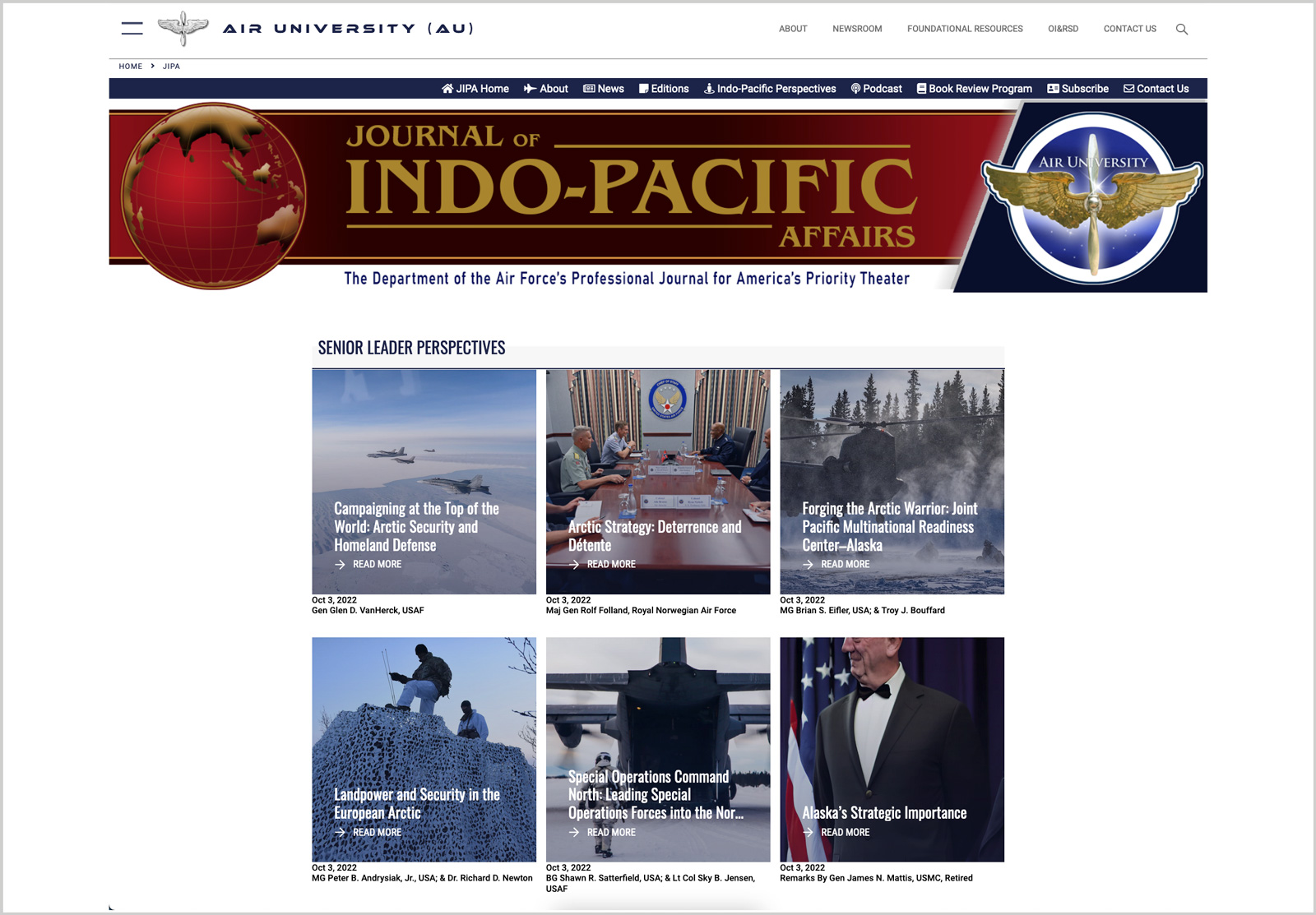The homepage of the Journal of Indo-Pacific Affairs (JIPA) features a sleek design with a symbol of wings over a propeller in gray on the left, representing the Air University (AU). To the right, the website displays navigational tabs including About, Newsroom, Foundational Resources, Cargo, Contact, and a Search bar marked by a magnifying glass. Additional menu items above include Home, About, News Editions, Indo-Pacific Perspectives, Podcasts, Book Review Program, Subscribe, and Contact Us.

Dominating the page is a large banner showcasing a red globe with the Asian continent highlighted, alongside the Air University emblem. The banner also introduces the Department of the Air Force's professional journal dedicated to America's priority theater with the title "Senior Leader Perspectives."

Below the banner, there are six clickable article boxes with titles such as:
1. Campaign at the Top of the World: Arctic Strategy
2. Forging the Arctic Warrior
3. Land Power and Security in the European Arctic
4. Special Operations Command North: Landing Special Operations Forces into the North
5. Alaska's Strategic Importance

The website invites readers to explore various resources and perspectives within the Journal of Indo-Pacific Affairs.